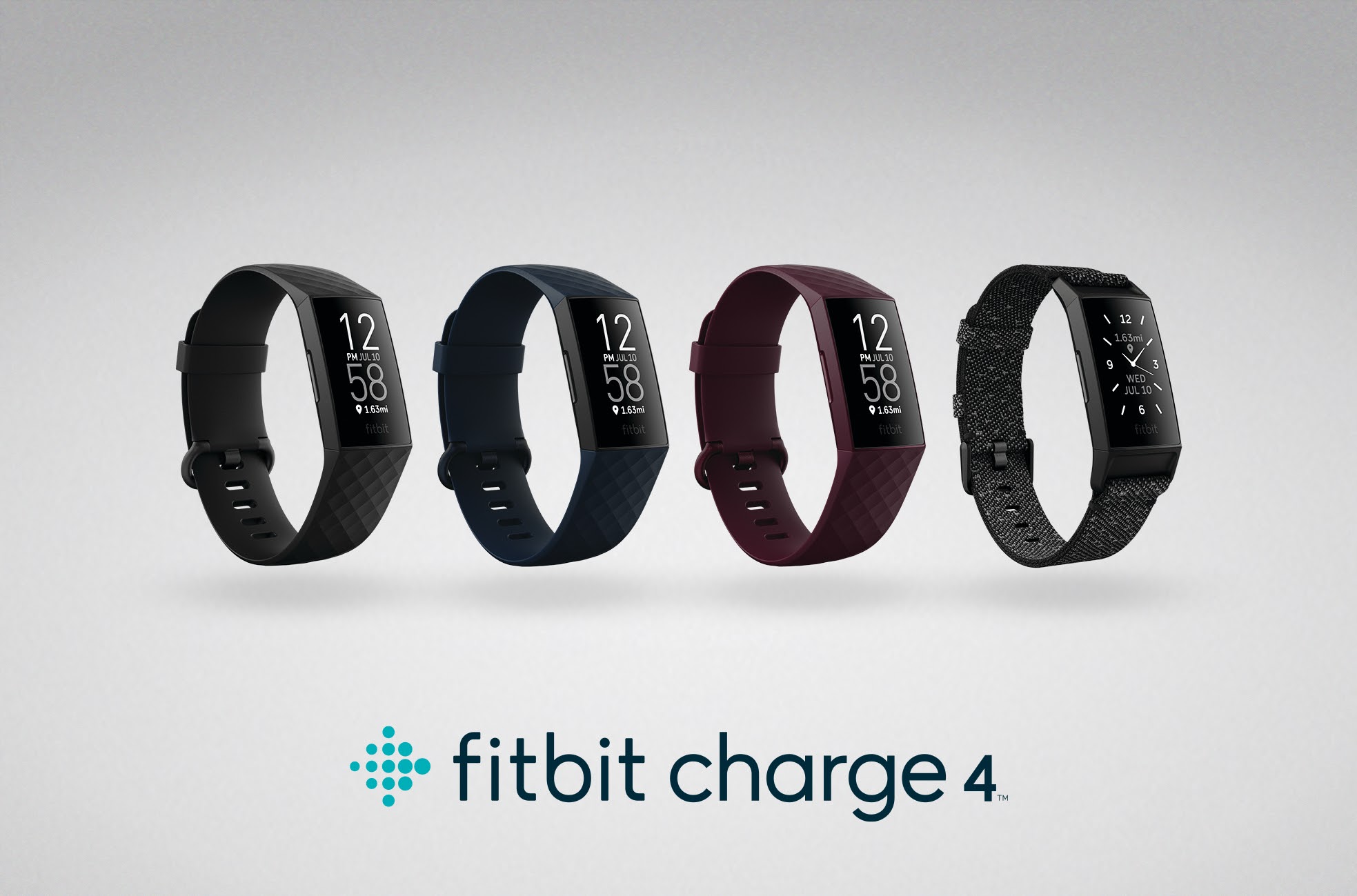The photograph showcases a collection of four Fitbit Charge 4 devices, prominently displayed at the top with the text "Fitbit Charge 4" in a sans-serif font at the bottom. The devices vary in color: two are black, featuring smooth and quilted designs, respectively, one is maroon, and the fourth, while also featuring a watch face with a leather wristband, stands out amidst the others. Each Fitbit has a rectangular screen, all displaying the numbers "12" and "58," which do not correlate with the actual time shown on the watch face (10:09). A tiny trademark symbol appears under the "4," and a series of gray circles forming a cross is visible near the Fitbit logo. The background is gray, highlighting the sleek and smooth exterior finishes of the devices.